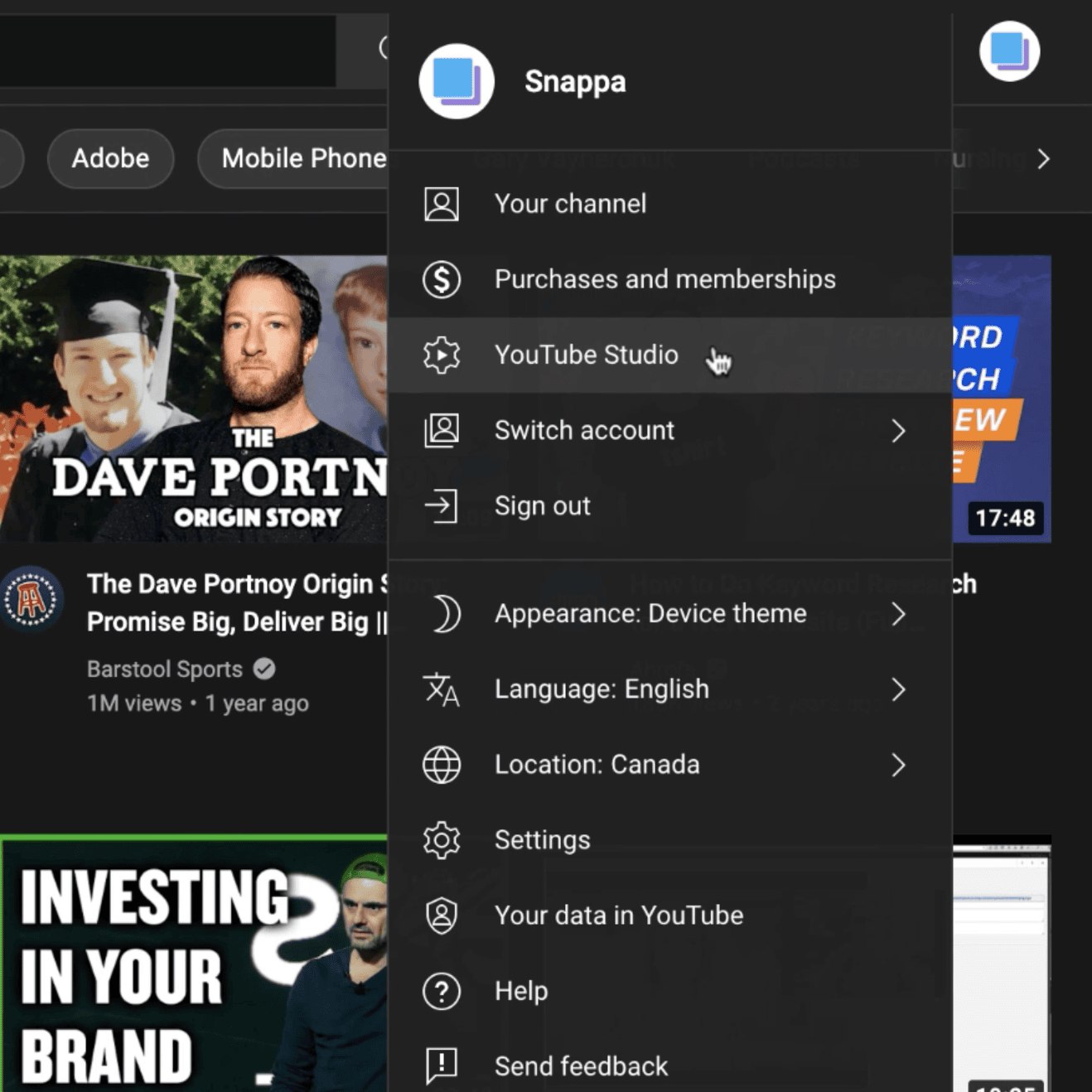Here’s a cleaned-up and more descriptive caption for the image:

---

The app page displayed belongs to Snappa, with a predominantly black background. Central to the display, a vertical menu spans from the top to the bottom. The menu itself also has a black background, harmonizing with the rest of the page. 

**Top Section:**
- At the very top right, there is a black search bar. Adjacent to it is an icon featuring a blue square in front of a purple square within a white circle.

**Mid Section:**
- Below this icon, dark gray buttons on the black background represent options for Adobe and mobile phone functionality. 
- The remainder of the background is mostly obscured by a pop-up window. However, certain elements are still visible:
  - To the far right of the background page, a white arrow indicates the option to navigate to the next page.
  - Below, in the background section, the headline "The Dave Portnoy Origin Story" is displayed in white text alongside three images of Dave Portnoy. The text is partially obscured, showing "Dave POR... Origin Story."
  - Another headline just below features an icon resembling a brown stool with white dots encircled in white. The visible text reads "The Dave Portnoy Origin S...". Right below, a slogan reads "promise big, deliver big."

**Further Down:**
- Additional text states "Barstool Sports" in grayish-white, followed by a grayish-white circle with a black checkmark, and the note "one million views · one year ago" in the same grayish-white text.
- A green bar appears beneath this, leading to an image of a middle-aged man in a green baseball hat. Accompanying text states "Investing in your brand" in white.

**Pop-Up Menu:**
- The pop-up menu in the middle starts at the top with Snappa's logo (a white circle with a blue square in front of a purple square). Beside it, the app's name “Snappa” is written in white.
- Below are the following options:
  1. **Your Channel:** Accompanied by a person icon.
  2. **Purchases and Memberships:** Featuring a dollar icon.
  3. **YouTube Studio:** Indicated by a gear icon with a play button inside.
  4. **Switch Account:** Marked with a person icon and an arrow for switching accounts.
  5. **Sign Out:** Denoted by an arrow icon.
  6. **Appearance:** Featuring a half-moon icon with the text “Appearance: Device Theme” and an accompanying arrow.
  7. **Language:** Indicated by a Chinese character icon with “Language: English” and an arrow.
  8. **Location:** A world icon with the text "Location: Canada" and an arrow.
  9. **Settings:** Shown with a gear icon.
  10. **Your Data in YouTube:** Displayed with a shield icon containing a person.
  11. **Help:** Featuring a question mark icon.
  12. **Send Feedback:** Marked by a speech bubble icon with an exclamation point.

**Lower Section:**
- On the background page, near the bottom, another Snappa icon is displayed, with a white arrow below it for page navigation.
- Below the icon, a large square occupies about a third of the page with a purplish-blue background. Text within the square shows dark blue with partially visible white letters: “R&D” and “C&H.”
- Further down, two orange icons with the white letters "EW" and "E" appear.
- The time 17:48 is displayed in white against a black background.

**Bottom Section:**
- The rest of the page includes indistinct sections, featuring black and gray bars, culminating in a timestamp presented in white on a black background, which is unclear due to size.

---